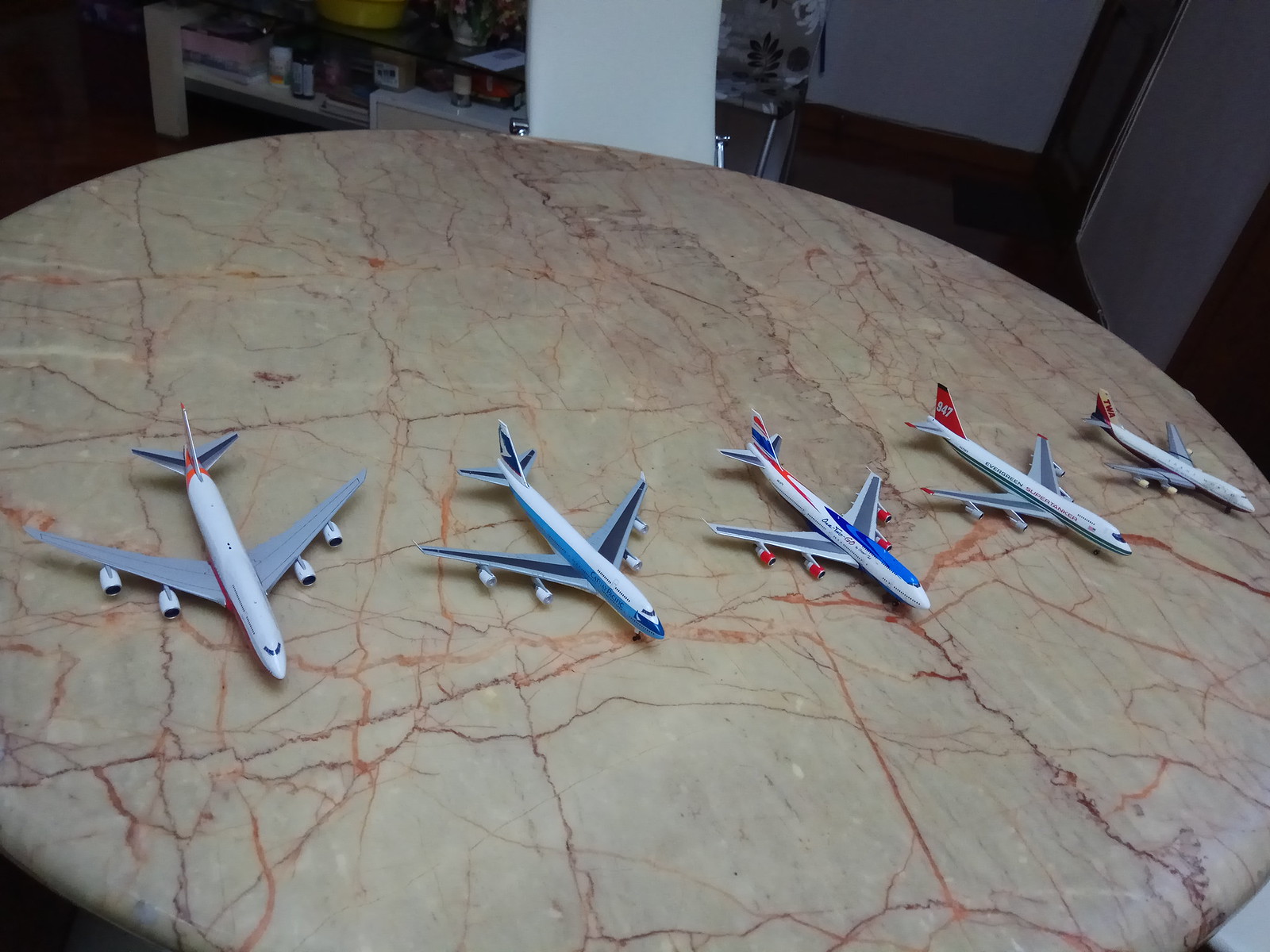The image is a square color photograph of a large, round, marble-like table with a beige hue, accentuated by veins of burgundy, reddish-orange, brown, and yellow. The table has noticeable stains of brown and yellow, adding to its intricate pattern. On top of this table are five scale model commercial airliners, likely made of metal and measuring approximately 8 to 10 inches in length. These miniature planes, representing different airline companies, feature predominantly white fuselages with gray wings and are arranged facing the bottom of the photograph, fanning out slightly to the right. The largest plane on the left has a red and blue tail, followed by one with blue, gray, and white colors, then another with red, white, and blue markings. The fourth jetliner sports a distinctive red tail, similar to a Virgin Airlines aircraft, while the smallest, fifth plane is white with gray wings and lacks visible text. The setting appears to be indoors, perhaps in a kitchen, partially revealing a white chair, metal shelves in a dimly lit background, and the hint of a hallway with white doors.